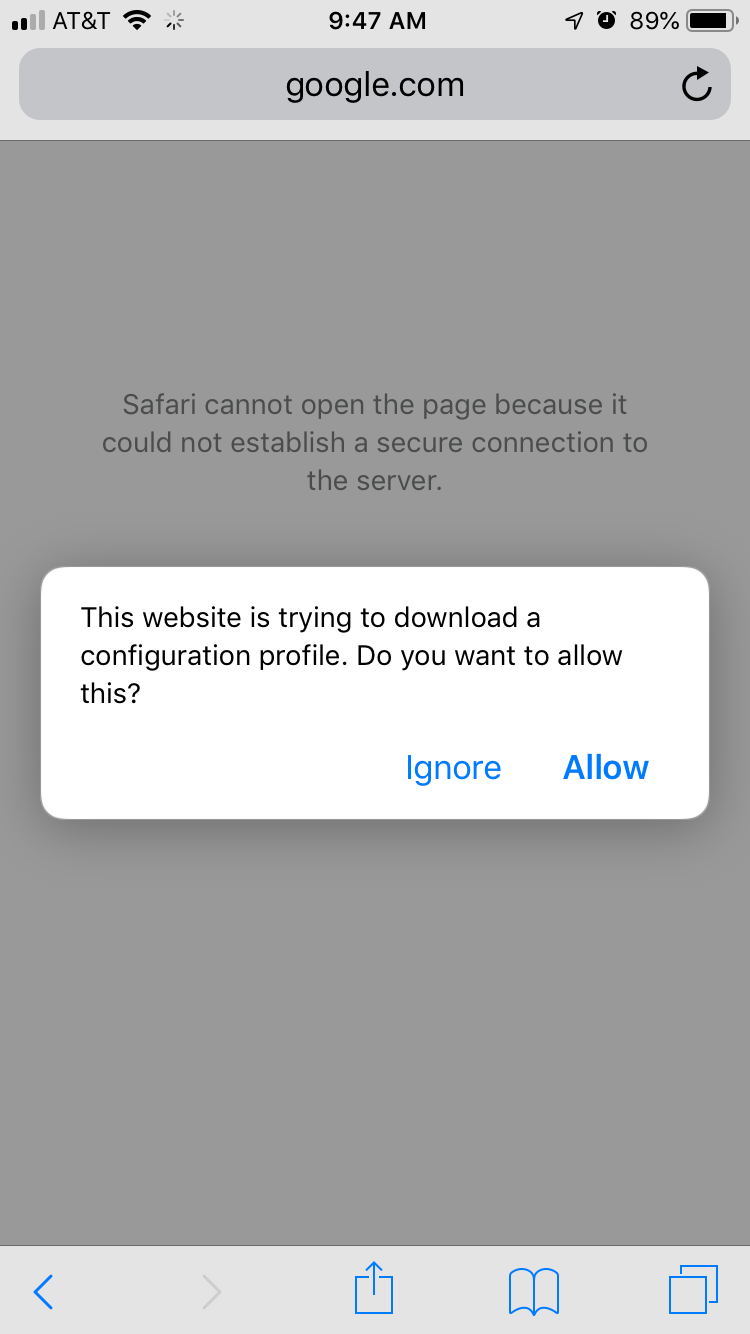The image depicts a smartphone screen, specifically captured at 9:47 AM, with these details visible:
- **Top Left:** Displays signal strength with 2 out of 4 bars, AT&T network, and full Wi-Fi signal.
- **Top Center:** Shows the time as 9:47 AM.
- **Top Right:** Battery level at 89%.
- **Browser Interface:** The screen shows a webpage open on Safari with the URL "google.com" and a refresh button. The search bar and navigation interface are in a gray theme.
- **Error Message:** A prominent message reads, "Safari cannot open the page because it could not establish a secure connection to the server."
- **Popup Notification:** Below the error message, there is a notification stating, "This website is trying to download a configuration profile. Do you want to allow this?" with options to "Ignore" or "Allow."
- **Bottom Navigation Bar:** Starting from the left, it contains a blue-back arrow, a square with an up arrow (likely for sharing options), and a book icon representing bookmarks. Additionally, there are two overlapping squares indicating open tabs.
- **Overall Theme:** The topmost part of the screen is gray, reflecting a maze-like pattern, and the interface indicates that this is a smartphone screen displaying a typical mobile web browsing session.